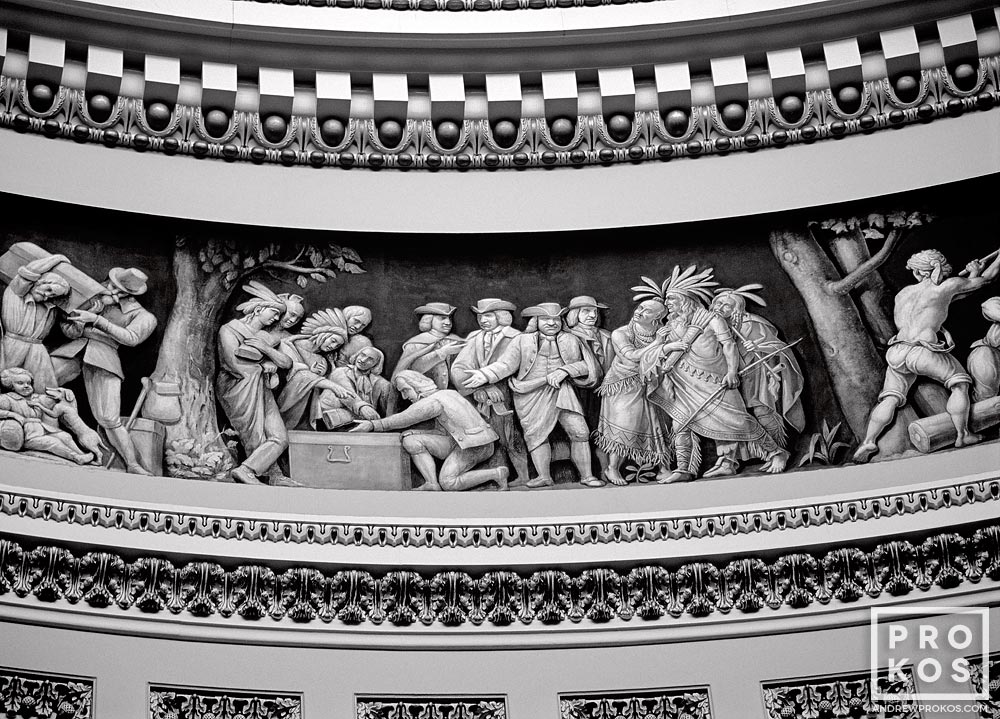The black and white neoclassical artwork, likely an ornate carving on the rim of a dome in a governmental building or an art museum, portrays a detailed scene of early interaction between pilgrims and Native Americans. Centered within the scene are various subjects, predominantly pilgrims, engaging in trade and negotiation over a table with the Native Americans, who are located more towards the sides. The focal point is a Pilgrim man extending his hand towards a box on the table, with his counterparts and a Native American chief, identifiable by his headdress, closely examining the contents. This central tableau is framed by two trees on either side; on the far right, a single pilgrim is seen pushing outward. On the far left, a small dog plays with a child, adding a touch of daily life to the historical narrative. Above and below this main depiction are intricate geometric patterns, featuring elements like spheres with a square nestled in a coat of olive branches, lending the entire piece an elaborate and cohesive aesthetic.